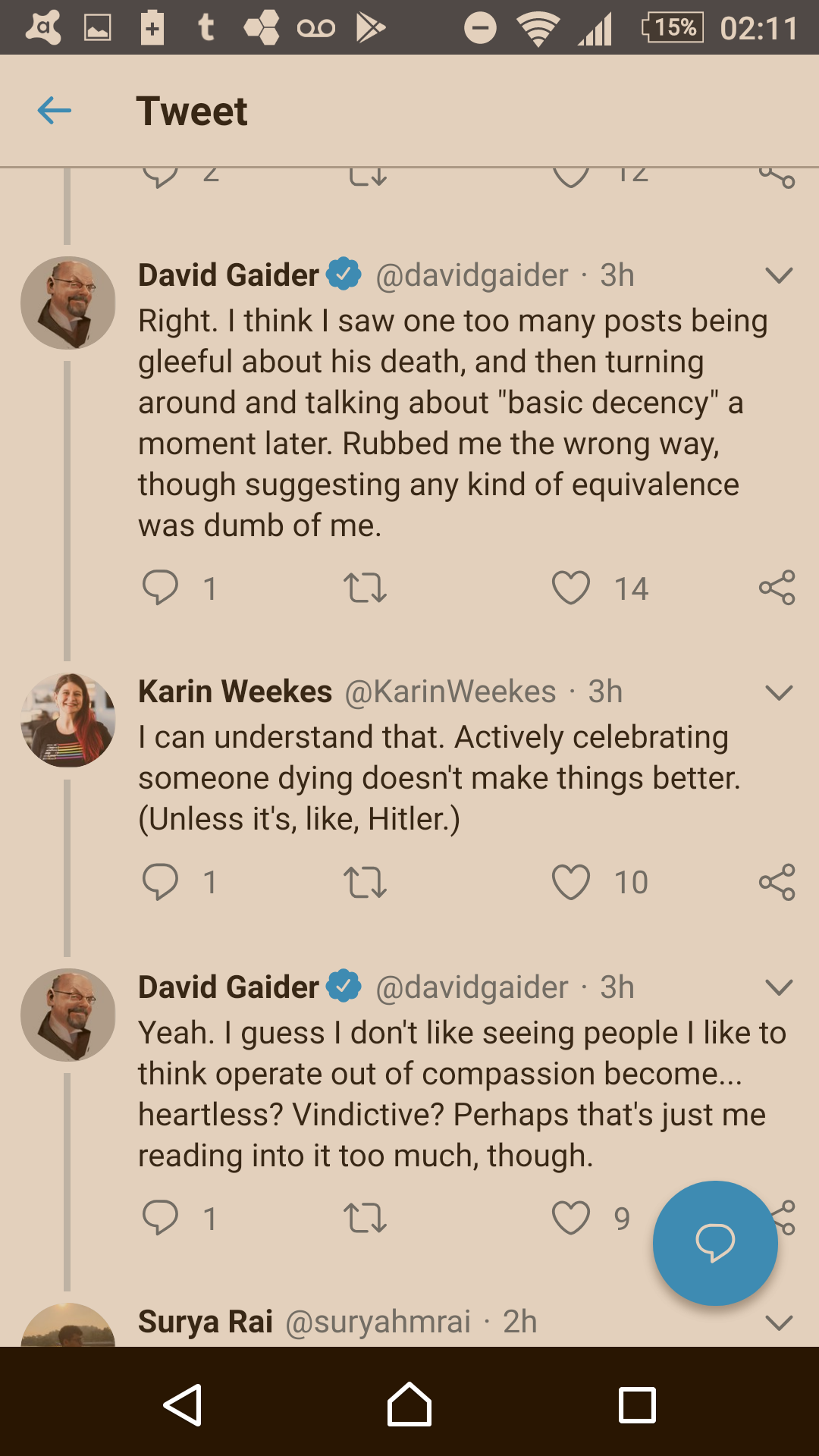Top left corner of the image contains various icons and symbols. There is a battery symbol with a plus sign indicating charge, the Twitter logo, and three shapes that could represent app icons. Additionally, there are circles, possibly representing settings or actions, and icons for the Play Store, Wi-Fi (full signal), cellular signal (full bars), and battery level at approximately 50%.

Towards the center-left, there is a greyed-out image indicating that the tweet it accompanies contains content that is obscured or hidden. Below this, the conversation in the image starts with a user named "divigator" who comments on the contradictory nature of celebrating someone's death and immediately transitioning to discuss basic decency. The response by "Karen Weeks" acknowledges the negative impact of celebrating death, except in extreme cases like Hillary Clinton, though she seemingly rebukes her previous stance.

Further into the conversation, divigator reaffirms their discomfort with people perceived as compassionate becoming heartless and vindictive, but also questions if they are over-interpreting the situation. Another user, "Syria Mirror," comments on the post, though their contribution is less clear due to the dullness in contrast.

The bottom part of the image features a black navigation bar with a left-facing triangle (likely a back button), a building icon (potentially representing an app or location), and a square (possibly the home button). The overall brightness of the image appears to be turned down.